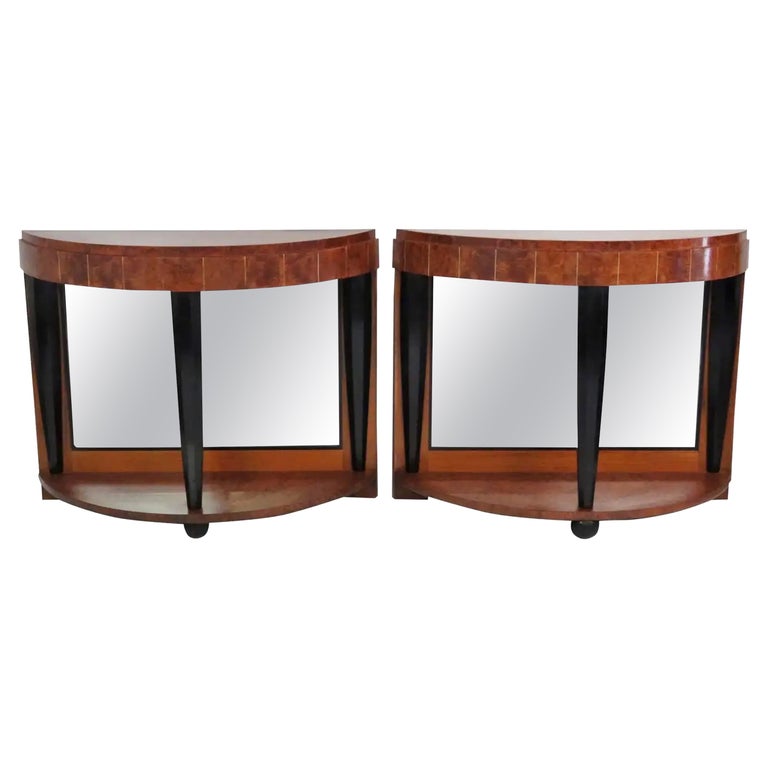The image displays a pair of modular semicircular tables positioned centrally against a plain white backdrop. Each table, constructed from a glossy, red cherry wood, resembles a horizontally sliced circle and, when combined, forms a complete circular table. The items together occupy a space about five to six inches wide and one and a half to two inches high in the photo. Both tables feature a flat back and gracefully curve forward into a half-circle shape at the front, creating an elegant visual effect.

The tabletop itself has a glossy finish and extends slightly beyond the underlying structure, adorned with a subtle quarter-inch edging which appears to be made of red-colored square tiles. Each segment of the round table is supported by three black-painted legs, performing both a structural and aesthetic role. The legs are anchored to semicircular black bases that add to the overall stability.

Moreover, between the legs, there's a light gray, possibly frosted glass or semi-transparent panel with a black frame, which adds a modern and sophisticated touch to the design. This panel bridges the space between the top and bottom surfaces of each table, providing additional functionality and reinforcing the stylish, finished appearance of the furniture.